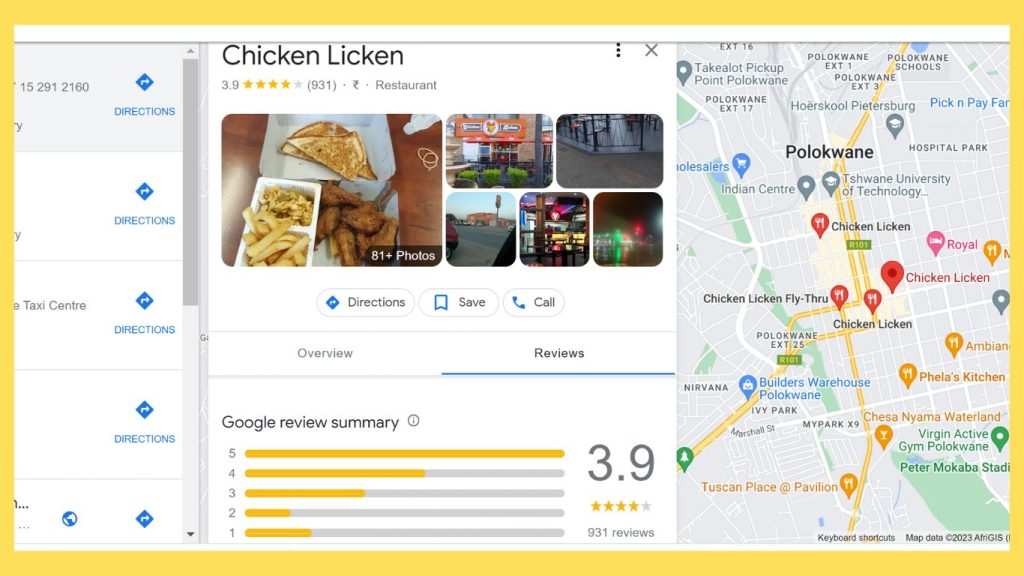The screenshot from Google showcases search results for a restaurant named "Chicken Licken." Prominently displayed at the top is the restaurant's name with a rating of 3.9 stars based on 931 reviews. The page appears to be under the 'Reviews' tab, showing a detailed breakdown of reviews by star rating, with the highest number of reviews being 5 stars, followed by 4, 3, 1, and 2 stars in descending order. Accompanying the text are a few images - one of a plated dish from the restaurant and another of the restaurant's exterior. On the right side of the screenshot, a map indicates the restaurant's location.